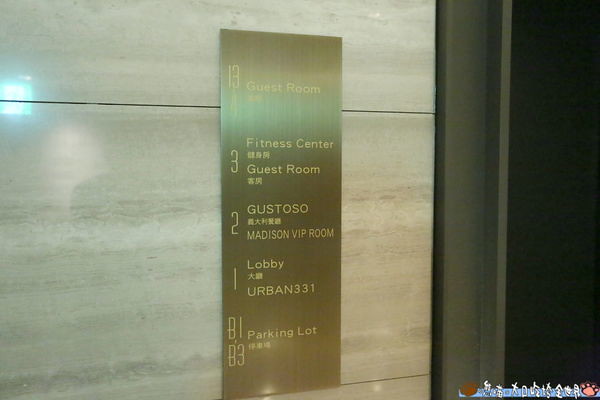The image depicts a vertically mounted, gold-toned metallic plaque on a grey marble wall, likely situated inside a modern building such as a hotel or office. The plaque, illuminated with white text, displays information about various floors and their corresponding facilities in both English and Chinese. Specifically, it lists: 13F Guest Room, 9F Fitness Center, 3F Guest Room, 2F Gustoso and Madison VIP Room, 1F Lobby and Urban 331, and B1 and B3 Parking Lot. The wall is made of large sections of grey marble with some dark trim on the right, potentially framing an entryway or elevator, suggesting the plaque is intended to guide visitors to their desired locations within the building.